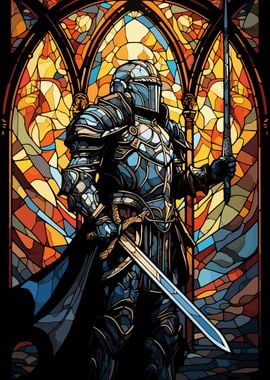A detailed stained glass illustration depicts an armored warrior, stylishly rendered with a comic book flair. The warrior is clad head-to-toe in intricate, steel-colored armor, complete with helmet, shoulder pads, and knee guards, evoking a medieval aesthetic. In the warrior's right hand, a sword points downward at a 45-degree angle, while in the left hand, another sword extends straight upward. 

The face is masked, obscuring any facial features, adding an element of mystery. The background showcases a vibrant stained glass window with arches and transepts, featuring an array of colors including red, blue, yellow, white, and subtle orange-brown hues. The glass is arranged in a pattern that resembles traditional church windows, enhancing the regal and historical feel of the image. The entire composition, rich in detail and color, creates a captivating and stylized representation of a majestic knight.